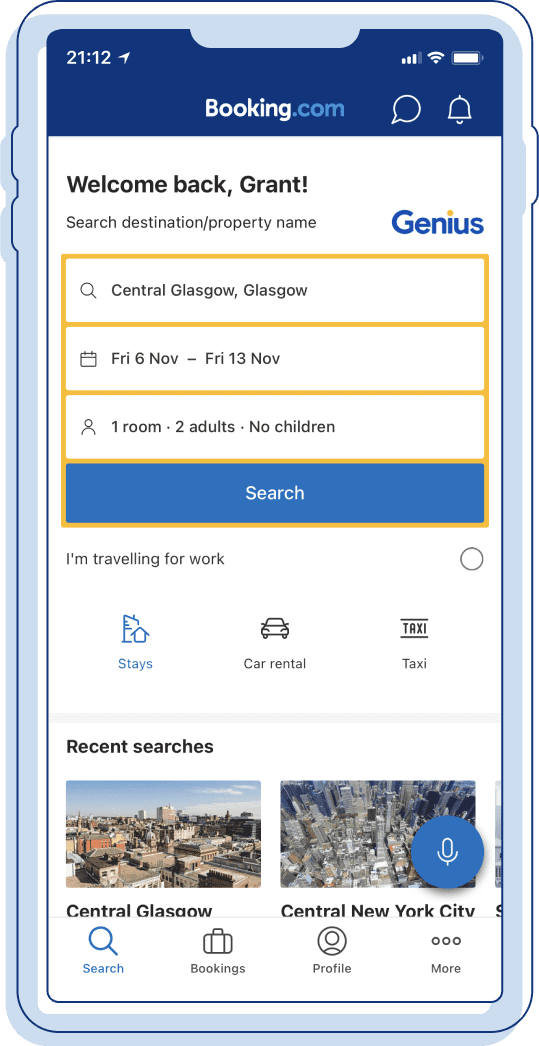This detailed illustration showcases a Booking.com graphic designed to promote their app. The image features a colored line drawing of a smartphone displaying the Booking.com app's homepage. 

At the top of the screen, the iconic Booking.com logo is prominently displayed. To its right, there are two white icons: a chat bubble and an alert symbol. The background below this header is a crisp white, featuring a bold greeting in black text, “Welcome Back Grant.” Below the greeting, a search prompt asks “Search Destination Property Name” to the left, while a large blue “Genius” text is on the right side.

The central section is divided into three rectangular boxes. The top box displays a search field set to "Central Glasgow." The middle box is a calendar field indicating a travel date from Friday, November 6th to Friday, November 13th. The bottom box specifies travel details: "One Room, Two Adults, No Children." A large blue search bar labeled “Search” in white text is situated directly below these boxes. Underneath the search bar, in small grey font, it reads, “I'm traveling for work,” accompanied by an unselected clickable button to the far right. 

At the bottom of the screen, three categories are centered: Stays, Car Rental, and Taxi, with Stays being selected. To the left of this section, under "Recent Searches," are two square photo thumbnails. The left thumbnail is labeled “Central Glasgow” and the right, “Central New York City.” A blue circular icon with a white microphone is positioned at the bottom right. 

Finally, the very bottom of the app interface features four icons: Search, Bookings, Profile, and More, providing easy navigation for users.